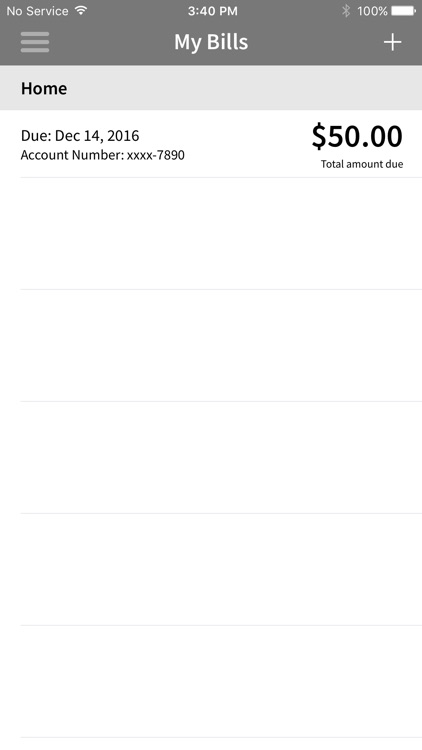This image is a detailed screenshot taken from a smartphone. At the top of the screen, there is a grayish banner with "No service" displayed in the left-hand corner. To the right of this, a fully connected Wi-Fi icon is visible. Centered at the top-middle of the image, the time is shown as "3:40 p.m." Moving further to the right, there is a slightly faded Bluetooth icon followed by a "100%" battery indicator and a fully charged battery icon.

Directly beneath this banner, to the left, there is a "hamburger menu" represented by three lines. Centrally located, the text "My Bills" is visible, and to the right of this is a plus sign. Below these, a gray rectangular banner houses the word "Home" aligned to the left.

The background of this section is predominantly white with segmented lines demarcating different areas. Only one section is filled in, displaying the following details: 

- "Due: December 14th, 2016"
- "Account Number: XXXX-7890"

Beneath these details, a large, bold, black text reads "$50." Following this, the text "Total Amount Due" is present. Various lines and spaces continue down to the bottom of the image, demarcating further sections that remain unfilled.